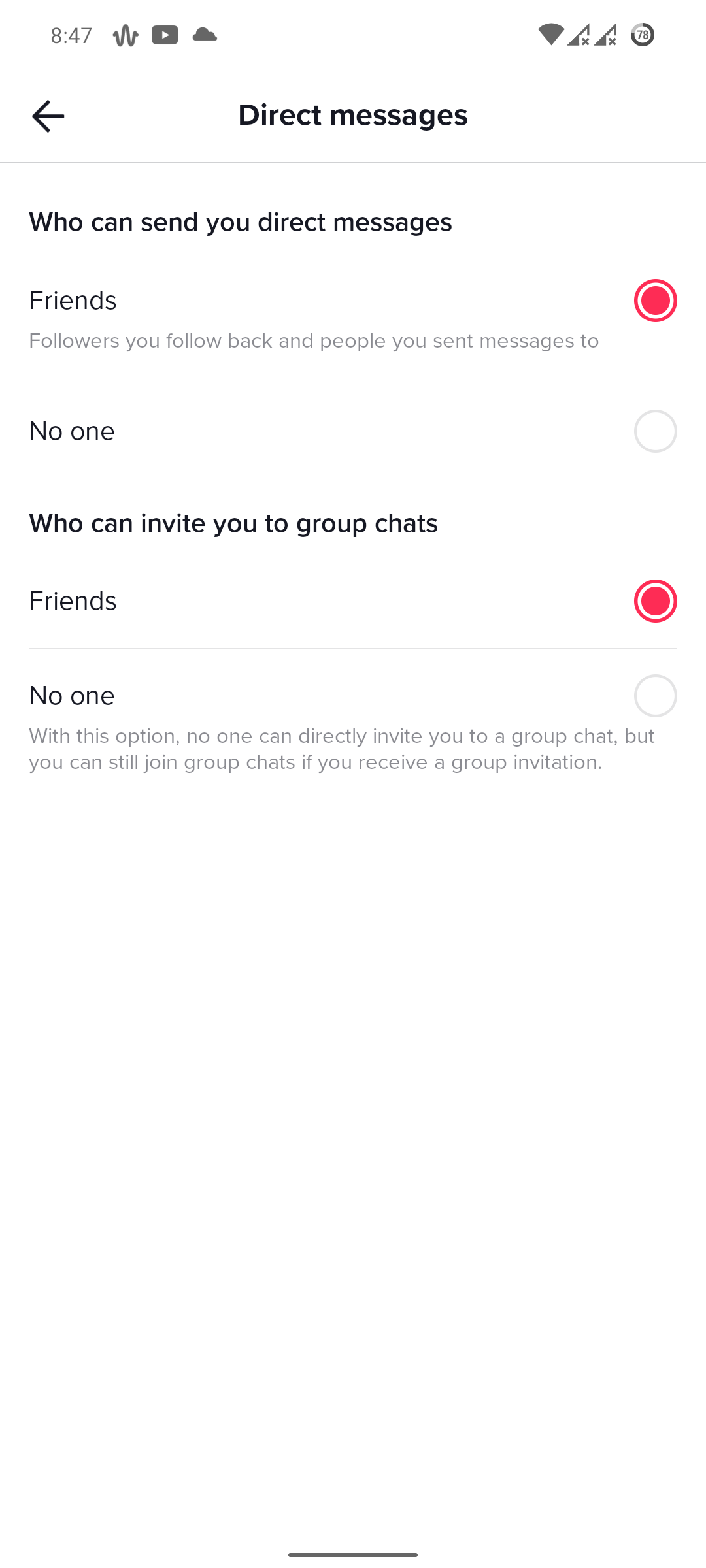This screenshot features an app interface displaying user settings for direct messages and group chat invitations. The top of the screen shows the current time, 8:47, along with several icons. From left to right, these icons include an unrecognized symbol, a gray box with a white triangle indicating a video play button, and a gray cloud icon. On the right side, there's an icon with a circle and the number 78, potentially indicating battery life.

The main section of the screenshot is set against a white background, with all text in black or gray shades. The prominently displayed header reads "Direct Messages" in black font. Below this, in a slightly lighter gray font, is the subheading "Who can send you direct messages." 

There are two options listed: "Friends" and "No one." The "Friends" option is marked with a red button, indicating it is selected. The "No one" option is represented by a clear, unselected gray circle with a white center.

Further down, a similar section titled "Who can invite you to group chats" is visible. The "Friends" option here is also marked with a red selected button, while the "No one" option is denoted by a clear, unselected gray circle with a white center.

This detailed configuration screen allows users to specify their preferences for receiving direct messages and group chat invitations, demonstrating a clear and user-friendly design.